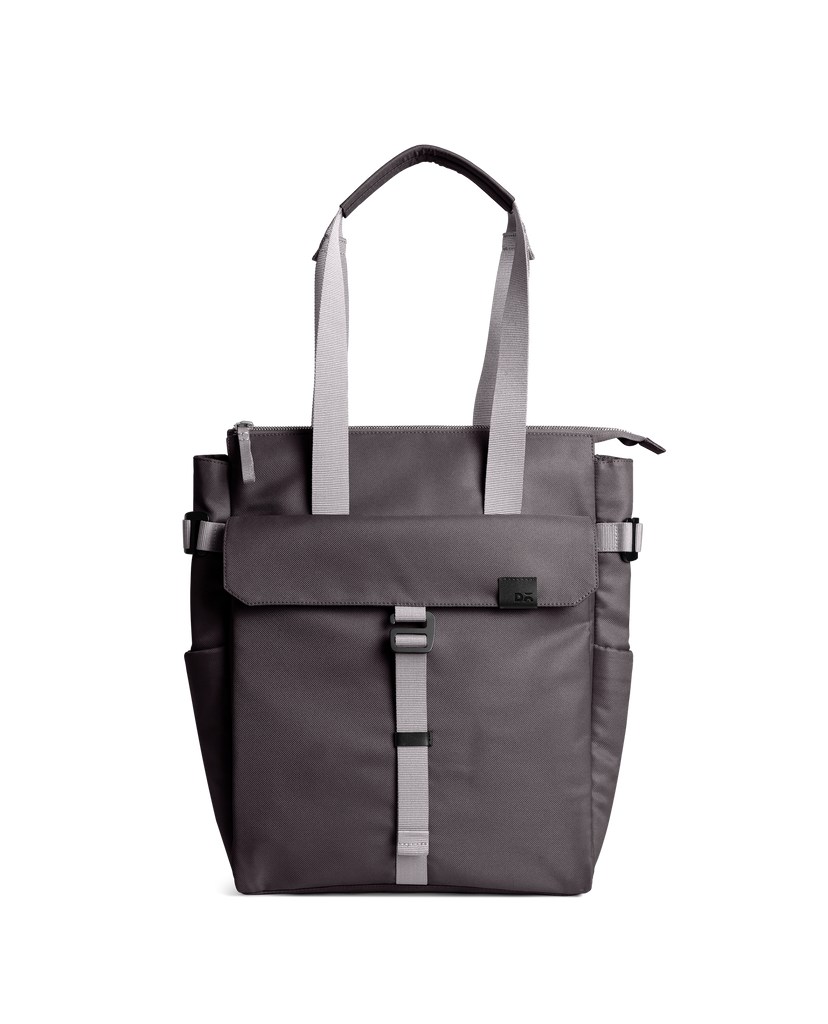The photograph depicts a utility-styled handbag composed primarily of dark charcoal gray with contrasting lighter gray straps. The main section of the bag features a robust central handle, padded in dark gray for additional comfort. The exterior is intricately designed, including an outer pocket secured with an adjustable strap and multiple attachment points for added functionality. One striking feature is a light gray strap that cascades down the center, leading to a flap above it, and a notable small black tab on the right side, useful for picking up the bag. The bag, potentially large enough to accommodate a laptop, also includes compartments and pockets, with a particular emphasis on a pocket that could easily store a water bottle. Additionally, there is a zipper on the left side, and the overall appearance is accentuated by a dark black tag, possibly inscribed with "DA." This comprehensive design makes it both practical and stylish. The backdrop of the photograph is white, which highlights the intricate details and diverse shades of gray on the handbag.